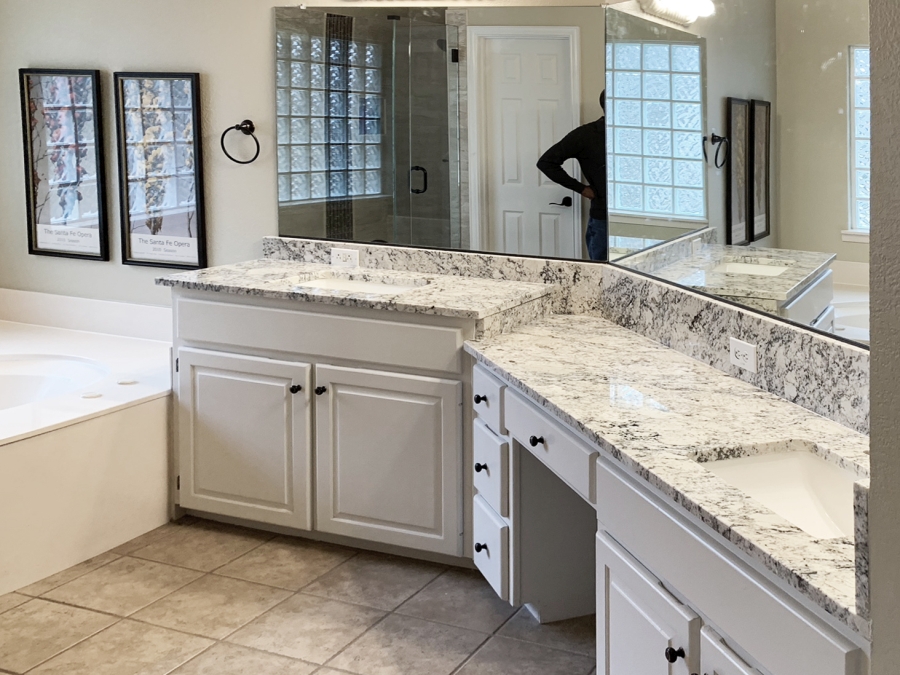This photograph depicts a spacious, modern bathroom, possibly a newly constructed display or a recently purchased home, as suggested by its pristine and unoccupied condition. The bathroom features two large mirrors mounted above marble countertops with small sinks and white-painted wooden shelves and drawers underneath for storage. Reflecting in the mirrors, we see a person wearing a black shirt standing between them, along with elements not directly visible in the image, such as a white doorway and a shower area. To the left, partially visible, is a bathtub adorned with two paintings on the wall above it and a towel rail positioned below the artwork and next to the first mirror. Two electrical outlets are situated above one of the sinks on the wall.